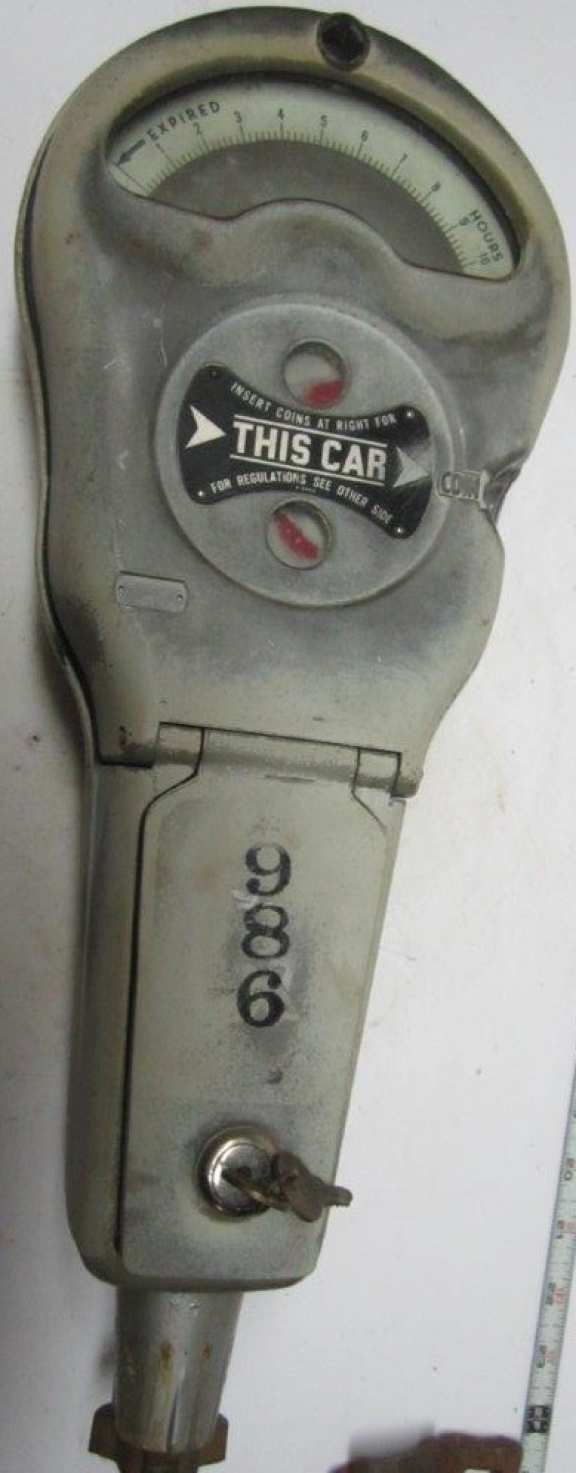The image is a tall, rectangular photograph featuring a very old-fashioned parking meter set against a white background. The meter is made of worn, grayish metal and is approximately 12 to 16 inches in height. Prominently displayed in the middle of the meter is a logo with the text "This car" flanked by arrows pointing in both directions, supposedly indicating where to park. Below this text, the numbers "986" are stamped, positioned above a key and lock mechanism typically used to access and empty the coins. Notably, there is a key inserted in the keyhole, with two keys attached to the key ring. A clear glass gauge at the top displays the amount of time remaining as coins are inserted. Additionally, next to the meter, on the lower right side of the image, there is a white measuring tape possibly used to indicate the dimensions of the object, which measures about two inches across and eight inches tall. Text on the meter directs, "Insert coins at right for this car. For regulations, see other side."